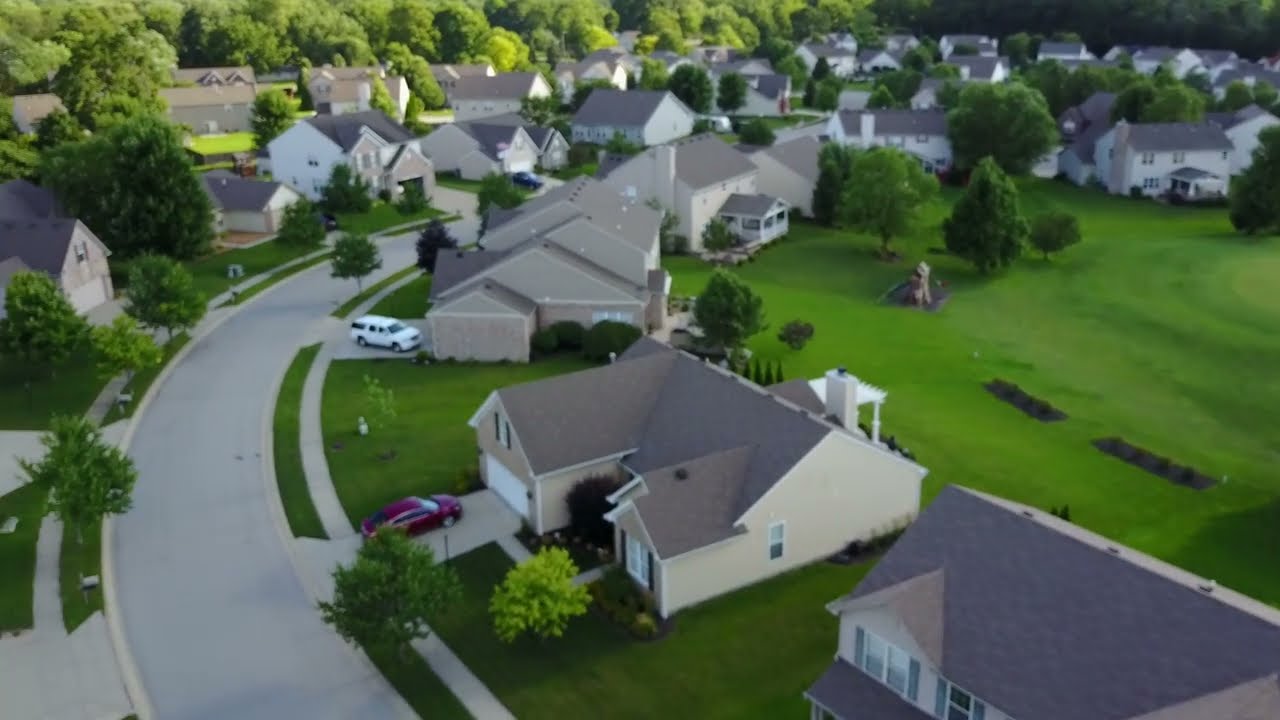The image is a detailed, realistic aerial drone photograph of a residential subdivision. In the foreground, two single-family homes stand side by side, each with distinctive features. The home on the left is a beige, split-level residence with a three-car garage, a small entryway, and a combination of brick facing on the lower portion and siding with navy blue shutters on the upper portion. It also has an American flag tied to one of the poles. The house on the right is a two-story structure with a two-car garage, gray siding, a dark-accented front, and brick facing. Both houses have triangular green roofs.

Between the houses, there is a row of large, lush trees, adding to the verdant scenery. These houses lead into a vast green garden area filled with vibrant grass and scattered trees. A pathway runs through the middle of this grassy field, and some vehicles are parked further back. In the background, another row of single-family homes, similar in style to the front ones, can be seen beyond the expansive lawn and trees. The entire scene is depicted with remarkable detail, making it almost indistinguishable from a drawn model.